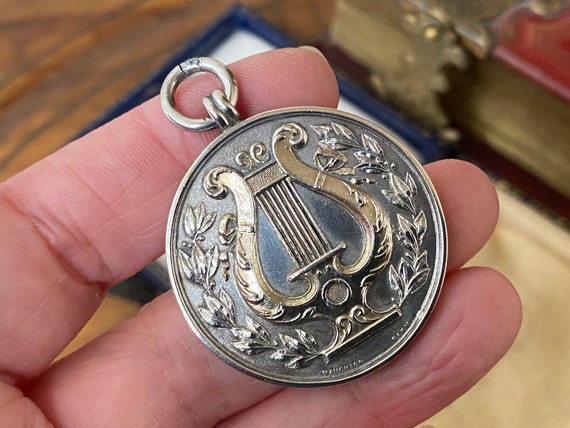The image depicts a Caucasian man's hand holding up a silver medallion, which has been fashioned into a necklace evidenced by a small bail at the top for attaching a chain. The man’s three fingers are prominently visible, supporting the medallion delicately. This piece, possibly a former coin or an award, is intricately stamped with a central lyre symbol flanked by wreaths, and has sections where the silver has a darker, almost golden hue, particularly on the lyre. The design is complex, featuring what appear to be flowers and coiled snakes on either side. In the background, blurred elements hint at a domestic setting: a red book extending out of the frame and a blue-outlined item that might be a box. This setting includes hints of yellow, white, light tan, and brown wooden flooring, suggesting the photo was taken indoors, possibly in a study or living room.